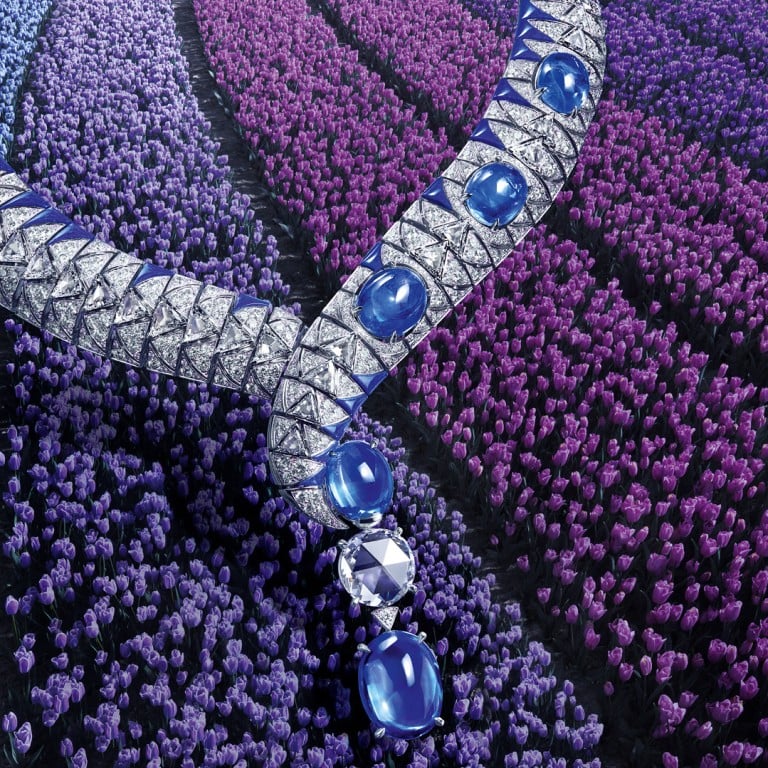This detailed photograph depicts a luxurious piece of jewelry, possibly a bracelet or necklace, artfully placed on an indigo-hued carpet. The carpet's fibers are exceptionally well-defined, showing various shades of purple and light blue, particularly accentuated in the top left corner. The jewelry itself, resembling silver snakeskin or diamonds, is intertwined with blue gems that line its right side. Toward its bottom part, the piece features a sequence of stacked jewels: a blue gem, a silver gem or crystal, followed by another blue gem. The image creates an illusion, making the jewelry appear almost larger than life, as if it were laid atop a field of vibrant purple flowers, adding to the deceptive yet captivating quality of this high-resolution shot.